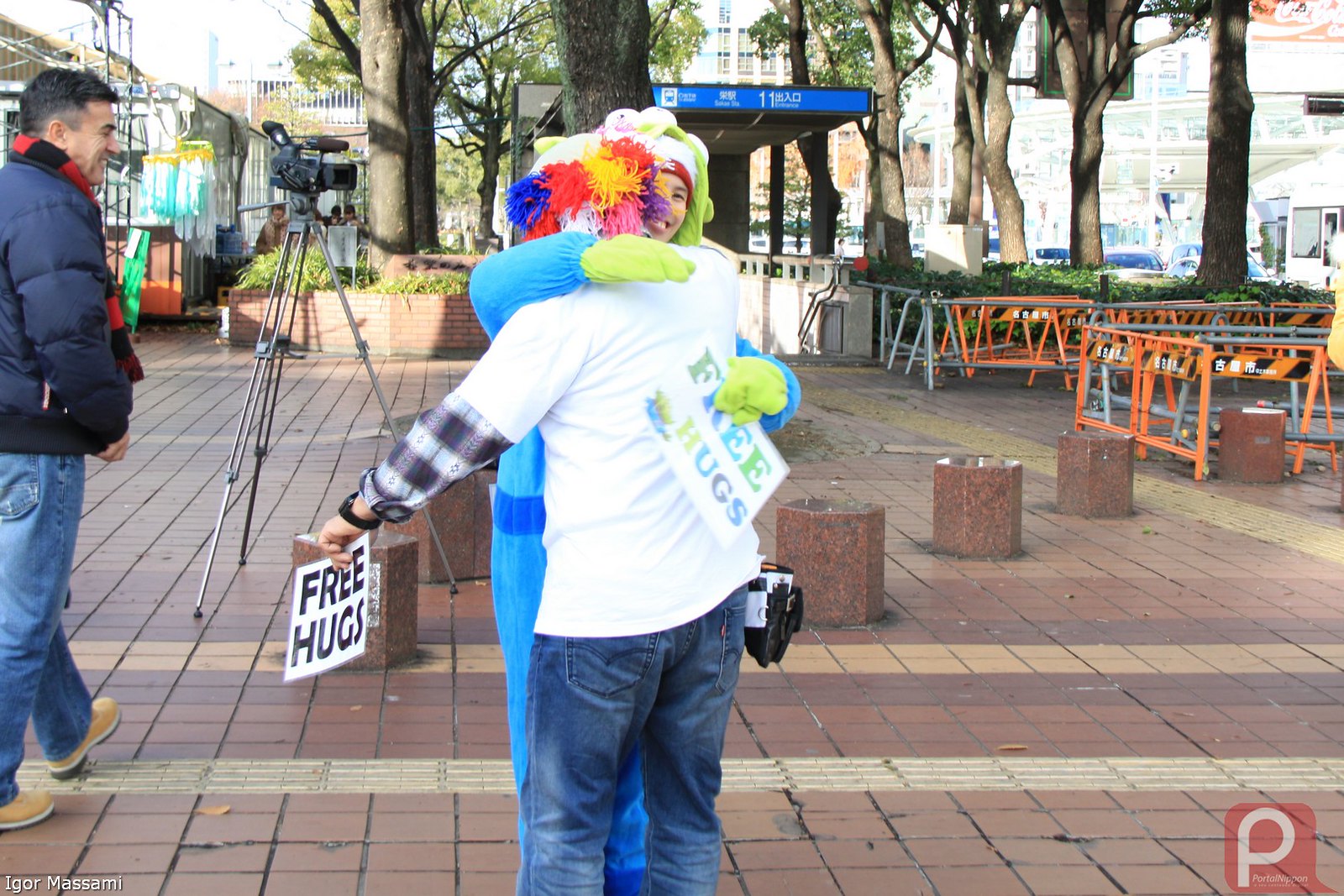In the image, two individuals are captured in a warm embrace on an outdoor walkway in what appears to be a vibrant city center or sidewalk fair. Both individuals, distinguishable by their distinct headwear adorned with funky colors and materials, hold signs proclaiming "Free Hugs." The scene features a woman dressed in a complete blue onesie and a man wearing a white t-shirt layered over a long sleeve shirt, paired with blue jeans. To their right, a passerby is seen laughing heartily at the sight of their affectionate display. Nearby, a camera is actively recording the interaction, suggesting a planned or spontaneous event aimed at spreading joy. In the backdrop, booths and chairs add to the fair-like atmosphere, enhancing the communal and lively spirit of the moment.